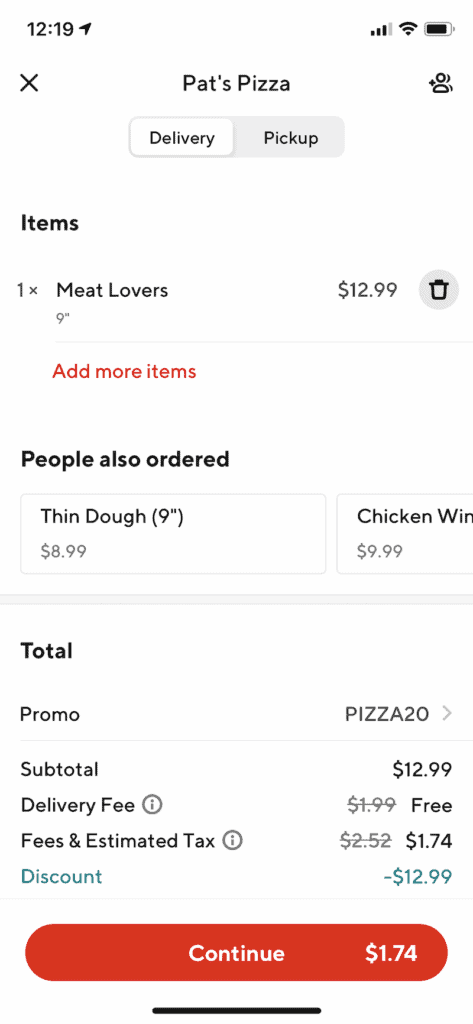This is a screen capture of a food delivery app, similar in design to Grubhub, featuring a clean, primarily white background with red accents. The most notable red element is a large "Continue" button positioned at the bottom of the page. The screen displays an ongoing delivery order from Pat's Pizza, with "Delivery" selected, indicated by a white button, while "Pickup" is grayed out. You can toggle between these options.

Listed under items, a "Meat Lovers" pizza priced at $12.99 is displayed, accompanied by a garbage can icon for item deletion. There is an option in red text to "Add more items," which is clickable. Below this, a black header reads "People also ordered," showcasing additional items that can be scrolled through horizontally. Visible options include "Thin Dough" and "Chicken Wings," priced at $8.99 and $9.99, respectively. However, the word "Wings" is partially cut off. 

At the bottom, there is a detailed price breakdown. A clickable promo code "PROMO PIZZA 20" is available for further details. The breakdown includes a subtotal of $12.99, a delivery fee listed as free with the original $1.99 stricken out, and fees and estimated tax initially $2.52, but reduced to $1.74. A discount of $12.99 is applied, highlighted in green. 

The final price of the order, an impressively low $1.74, is prominently displayed to the right of the "Continue" button.